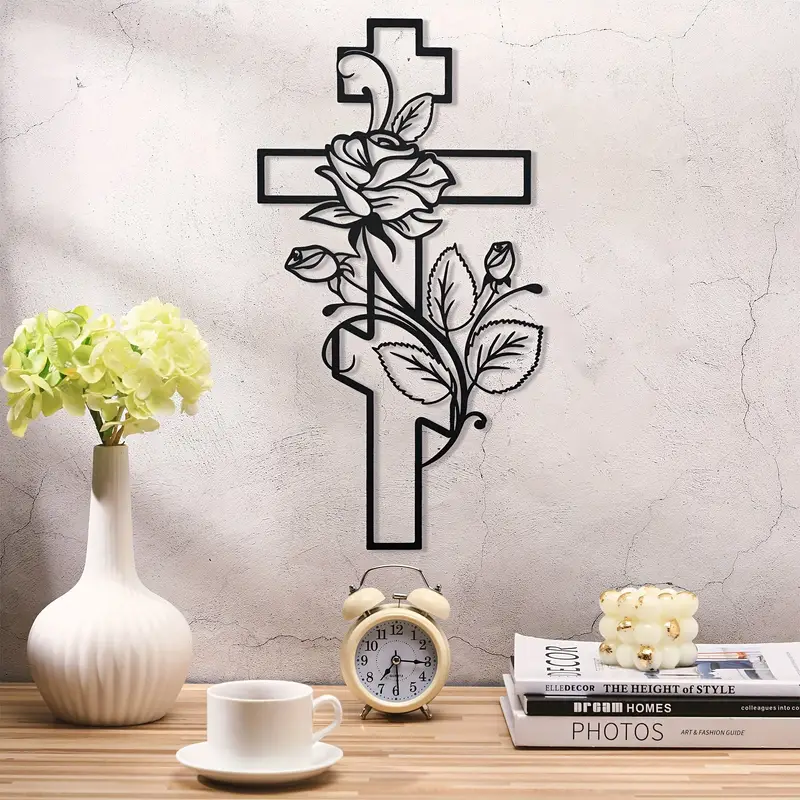The photograph showcases an indoor setting with a light beige wooden desk or shelf against a gray, cracked wall. Central to the image is a small, cream-colored analog alarm clock indicating 7:30, positioned on the desk. To the right of the clock is a stack of several books, topped with a small, cream-colored paperweight. Adjacent to the clock on the left is a white coffee mug resting on a matching white saucer. Further to the left, a white or cream-colored vase holds a delicate arrangement of greenish-yellow and whitish flowers. Dominating the wall above the desk is an intricate black metal wall hanging shaped like an Orthodox cross. This cross features a horizontal line at the top and a diagonal line at the bottom, adorned with a vivid floral design of roses and leaves weaving through its structure. The cross casts a noticeable shadow, adding depth to the wall's texture.